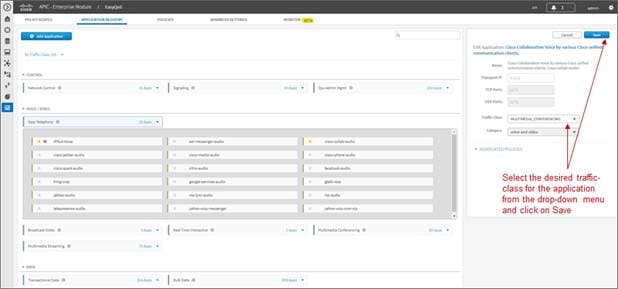The image appears to be a blurry screenshot of a user interface.

At the top of the screen, there is a dark blue or black banner featuring white text positioned on both the upper left and right corners. On the right side within this banner, a white box can be seen, presumably containing a notification bell icon. 

Along the left edge of the screen, there is a light gray vertical bar displaying various icons. From top to bottom, these icons likely represent Home, Files, and a blue box at the bottom, which could signify a different section or function.

Towards the upper left corner of the main section of the interface, there is a blue button accompanied by a block of small black text immediately to its right. The remaining space to the right is predominantly white and open.

Below this section, there is a table set against a light gray background. The table consists of three columns, each comprising six white rectangular boxes. 

At the bottom of the table, there are two lines of black text, which might provide additional information or context related to the table's content.